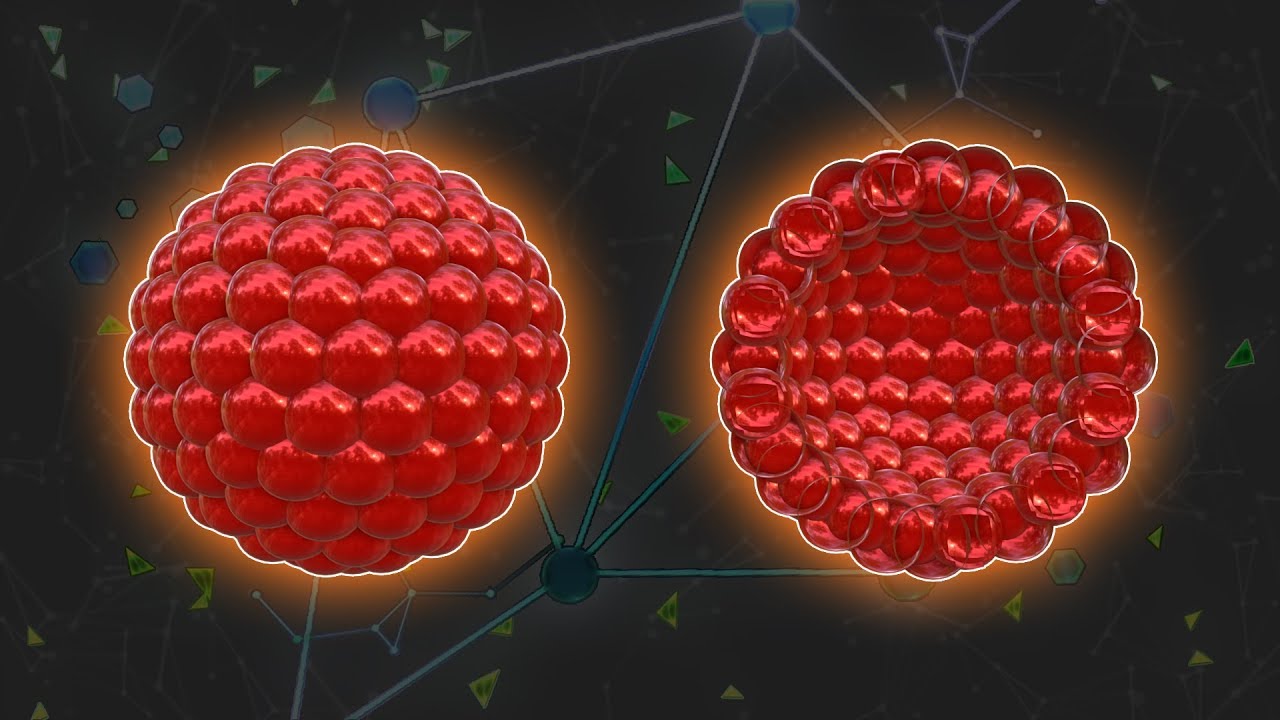This is a horizontally aligned rectangular computer-generated image with a dark background that features numerous small, green triangles and a few floating hexagons in blue and green. The focal point is two large circular objects situated in the center. The object on the left is a solid dome shape resembling a large raspberry, composed of clustered red, shiny orbs with gold flickers. The object on the right appears as if it has been sliced open, revealing its hollow interior made up of similar red orbs. Gray lines, which evoke an atomic or scientific aesthetic, connect various shapes, giving the impression of interconnected elements. The overall image conveys a scene that could fit within a video game or a scientific visualization, emphasizing a blend of geometric forms and organic-like structures.